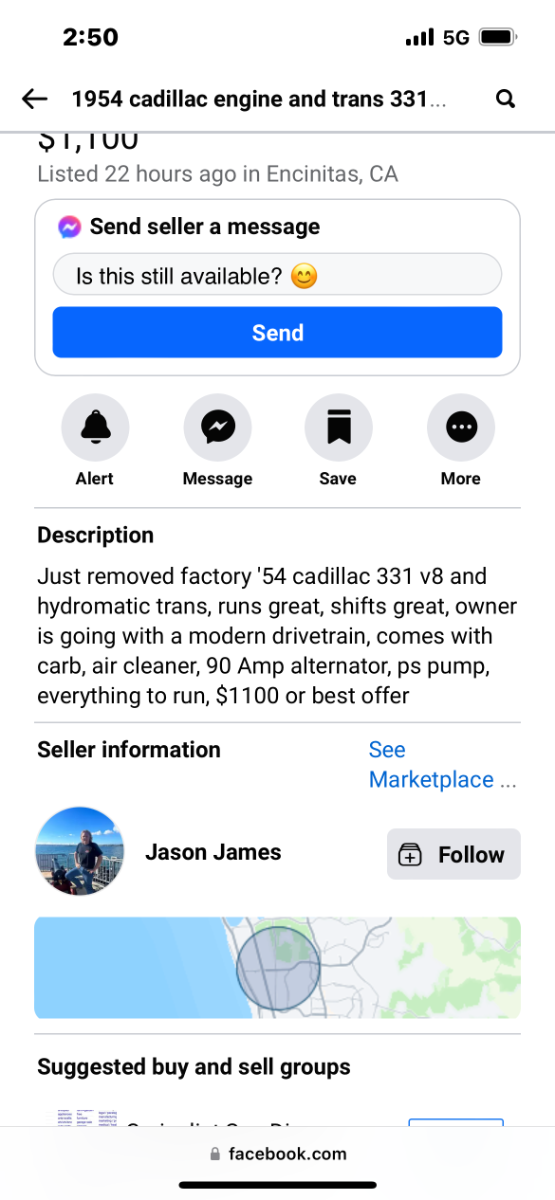**Detailed Caption:**

A screenshot displaying a Facebook Marketplace listing on a mobile phone. The time in the top status bar is 2:50 PM, accompanied by a full 5G service indicator and a full battery icon. The content header reads "1954 Cadillac Engine and Trans 331," flanked by a back button on the left and a search button on the right.

The listing details reveal the asking price of $1,100, noted as being posted 22 hours ago in Encinitas, California. Available interaction buttons include "Send Seller a Message" with the prompt "Is this still available?" and a send button beneath it. Additional buttons for alert, message, save, and more follow below.

The description reads: 
"Description: Just removed factory '54 Cadillac 331 V8, Hydramatic trans, runs great, shifts great, owner is going with a modern drivetrain. Comes with carb, air cleaner, 90 amp alternator, PS pump, everything to run. $1,100 or best offer." 

Seller information is displayed, listing Jason James as the seller, with a map of his location and options to follow him or see more marketplace listings. The footer of the phone UI shows "facebook.com" with a secure connection indicator.